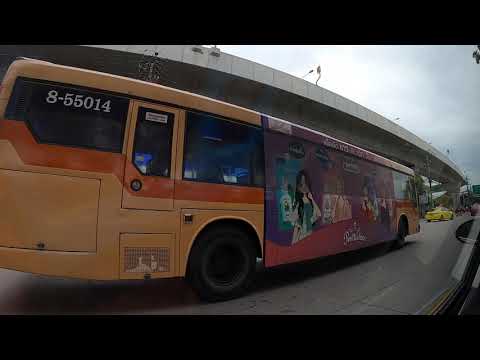The image is a horizontally-oriented, close-up photograph of a large city bus. The bus is primarily yellow with a bright orange stripe down the center and various decorations and advertisements along its midsection, featuring children's faces and what appears to be women dressed in dresses, though the details are blurry. The bus has the number 8-55014 displayed on both a side window and the back. A conspicuous yellow taxi is positioned in front of the bus, indicating that the bus is either parked or moving slowly down a city street. The image includes thick black borders at the top and bottom, and the setting features a gray, cloudy sky with bright white clouds in the upper right corner. Additionally, an overpass curves around to the left above the bus, contributing to the urban environment of the scene. The photograph seems to be taken from the perspective of another car's window.